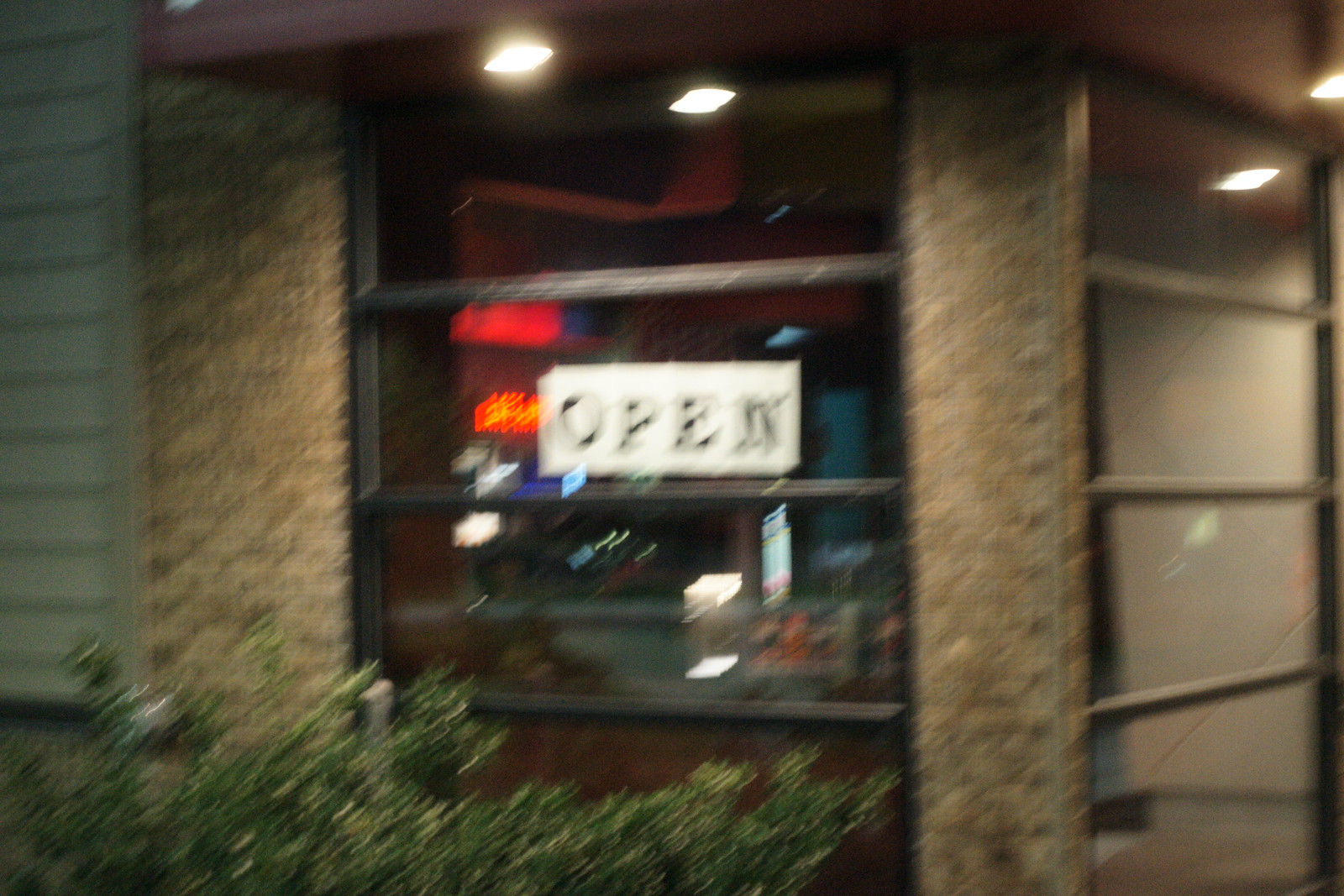A blurry nighttime photograph captures the exterior corner of a business establishment. The scene is set on a sidewalk bordered by green bushes and other landscaping elements. The building's facade features large glass windows, prominently displaying a white sign with black letters that spell "Open." A stone or light brown brick column marks the corner of the structure. Inside, vibrant red neon lights adorn the walls, contrasting with additional white neon lights positioned lower down. The reflection of a flat-screen TV adds a modern touch to the interior's illuminated ambiance.